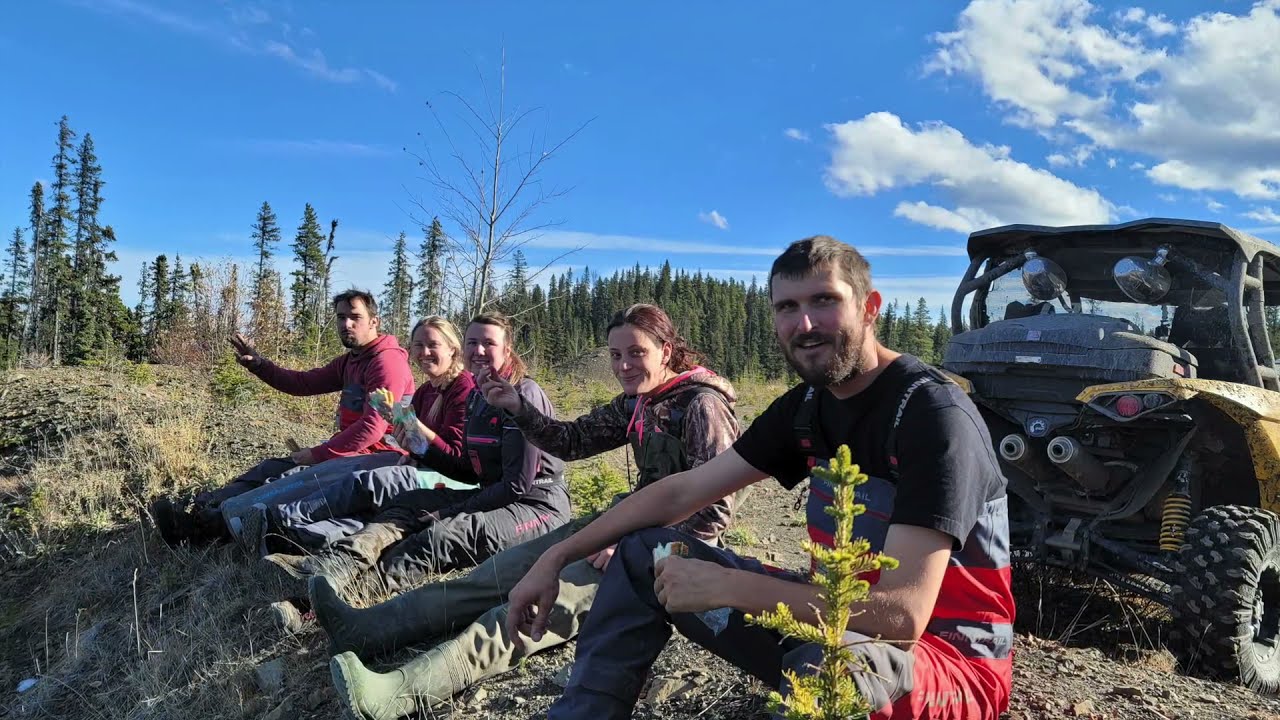In this vibrant outdoor photograph, a group of five friends is captured sitting on a rocky, dirt-strewn hill amidst a forest clearing. All smiles, they seem to be enjoying a sunny adventure day. Surrounding them are towering pine and evergreen trees set against a crisp blue sky dotted with a few clouds. The friends appear relaxed and casual in their outdoor attire, which ranges from t-shirts and long sleeves to camo clothing and a burgundy hoodie. The first man on the left, who sports a beard and short blonde hair, is dressed in red-striped overalls over a black t-shirt. Next to him, a woman clad in a dark sweatshirt with pink drawstrings and mud boots holds something small, likely a snack. Two more women beside her, one enjoying a sandwich and another in camo, are followed by a slightly overweight man at the end doing a peace sign, also dressed in a burgundy hoodie. Set slightly behind them to the right is a rugged, yellow side-by-side off-road vehicle, clearly marked by its distinct absence of fenders, chunky knobby tires, yellow springs, and dual metal tailpipes. The friends' joyful demeanor and the unique vehicle suggest they're amidst an exhilarating off-road trail adventure.